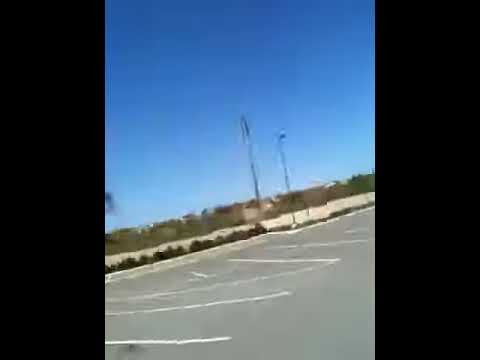The image depicts a grainy, low-resolution photograph of a standard parking lot, characterized by significant compression artifacts. The lot is covered in black pavement with white lines designating parking spaces, which appear jagged due to the image's poor quality. Flanking the parking area are green bushes, and beyond that, a white fence or wall. Two tall lampposts, presumably for nighttime illumination, are visible. In the background, a ridgeline filled with green trees can be seen. The sky above is a vivid blue, completely clear without any clouds. There are no people or cars present in the parking lot. Notably, the image features thick black bars on the left and right sides, suggesting it might be a still frame from a video.